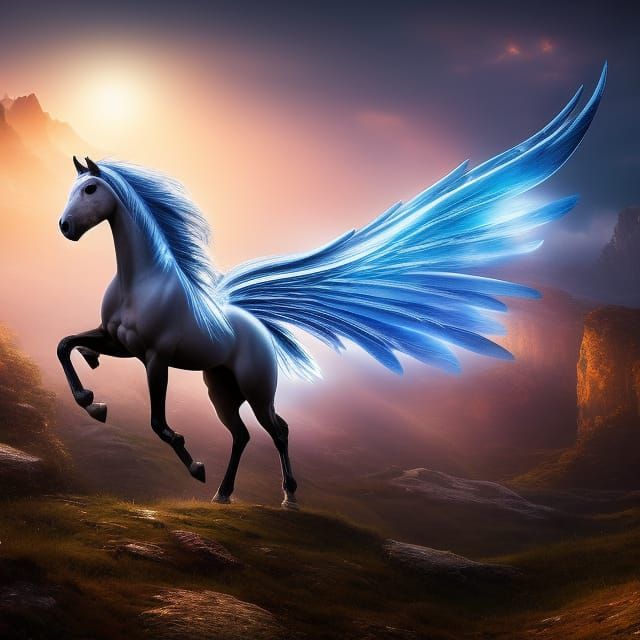This detailed digital rendering depicts a majestic Pegasus rearing up against a dimly lit, rocky terrain. The fantastical creature, boasting bold, blue luminescent wings and a flowing blue mane and tail, stands out strikingly against the background. The scene, possibly AI-generated due to noticeable rendering flaws like duplicated and improperly rendered legs, captures the Pegasus with its front legs dramatically outstretched and wings spread wide, basking in a curious blend of natural and ethereal light. The dimly lit, hilly, or mountainous surroundings are intermittently illuminated by what appears to be a surreal yellow beam of light, giving the impression of either a rising or setting sun, though the overall darkness suggests a nighttime setting. This blend of realistic and fantastical elements creates a captivating yet slightly disconcerting image, reminiscent of 1980s airbrushed van art.